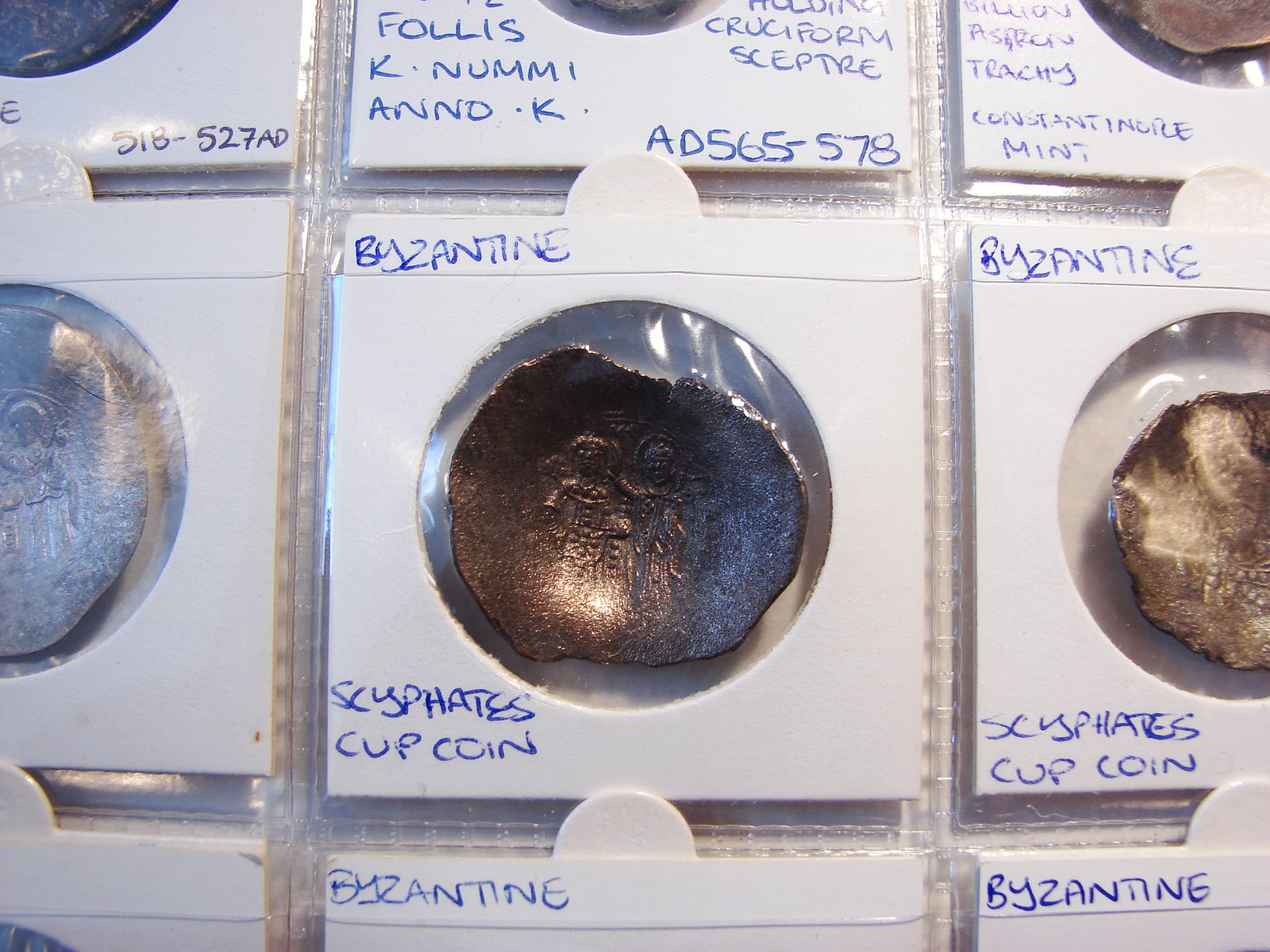The photograph depicts an ancient coin housed within a white, square packet. This packet features a circular, transparent plastic window at its center, revealing the coin inside. The coin itself is a dark brown, hammered piece with jagged and chipped edges, adorned with faint line drawings of people. The packet is labeled with blue handwritten text, with "Byzantine" inscribed at the top and "Socrates Cup Coin" at the bottom. The image is focused on this central coin, while other similar packets, each containing different ancient coins, are partially visible around the main packet. These surrounding packets also bear blue handwritten labels and are organized in a binder-like arrangement, suggesting a collector's display. Some of these additional packets include lighter gold and silver coins, hinting at a varied collection.